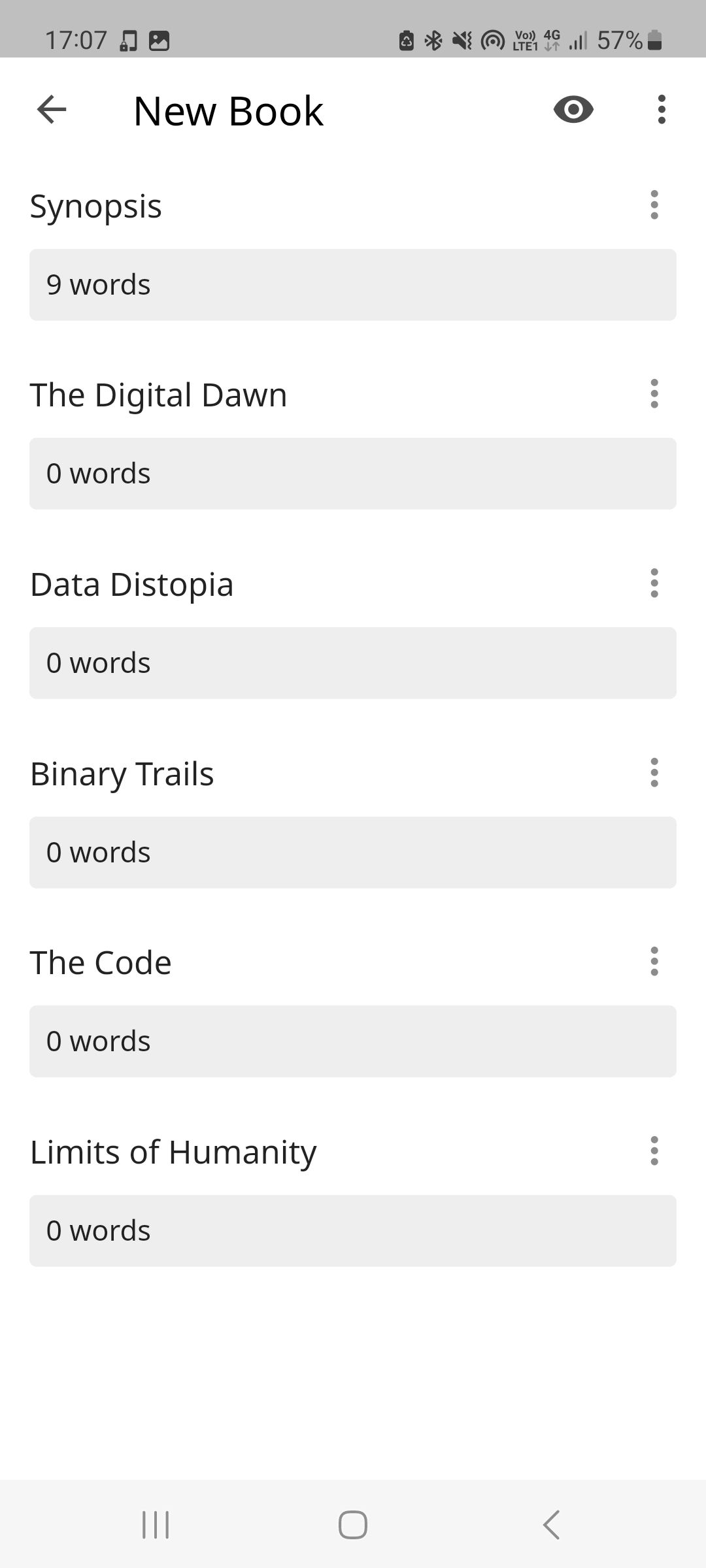In this image, the background is a light purple hue. At the very top of the screen, the time is displayed as 17:07, with a 57% battery indicator to its right. Below, there is a white horizontal bar featuring a left-facing arrow icon followed by the text “New Book”. To the right of this, there's an icon resembling the CBS eye logo, accompanied by a cluster of three small dots.

Beneath this white bar, there is a series of purple boxes. The first purple box contains the text "Synopsis" with three dots to the right of the word, hinting at additional options. Following this are multiple purple boxes, labeled with different topics. The first purple box contains nine words, with the title "Digital Dawn" and three dots next to it. The subsequent purple boxes have no words but are each titled and accompanied by three dots: "Data Dystopia," "Binary Trails," "The Code," and "Limits of Humanity."

At the bottom of the image, another purple box appears, this time featuring three horizontal lines, a square, and a left-facing arrow.

The overall impression is that this image outlines sections of a new book, offering a synopsis and different thematic chapters or sections such as "Digital Dawn" and "Limits of Humanity," each potentially with additional options for details or actions denoted by the accompanying three dots icons.